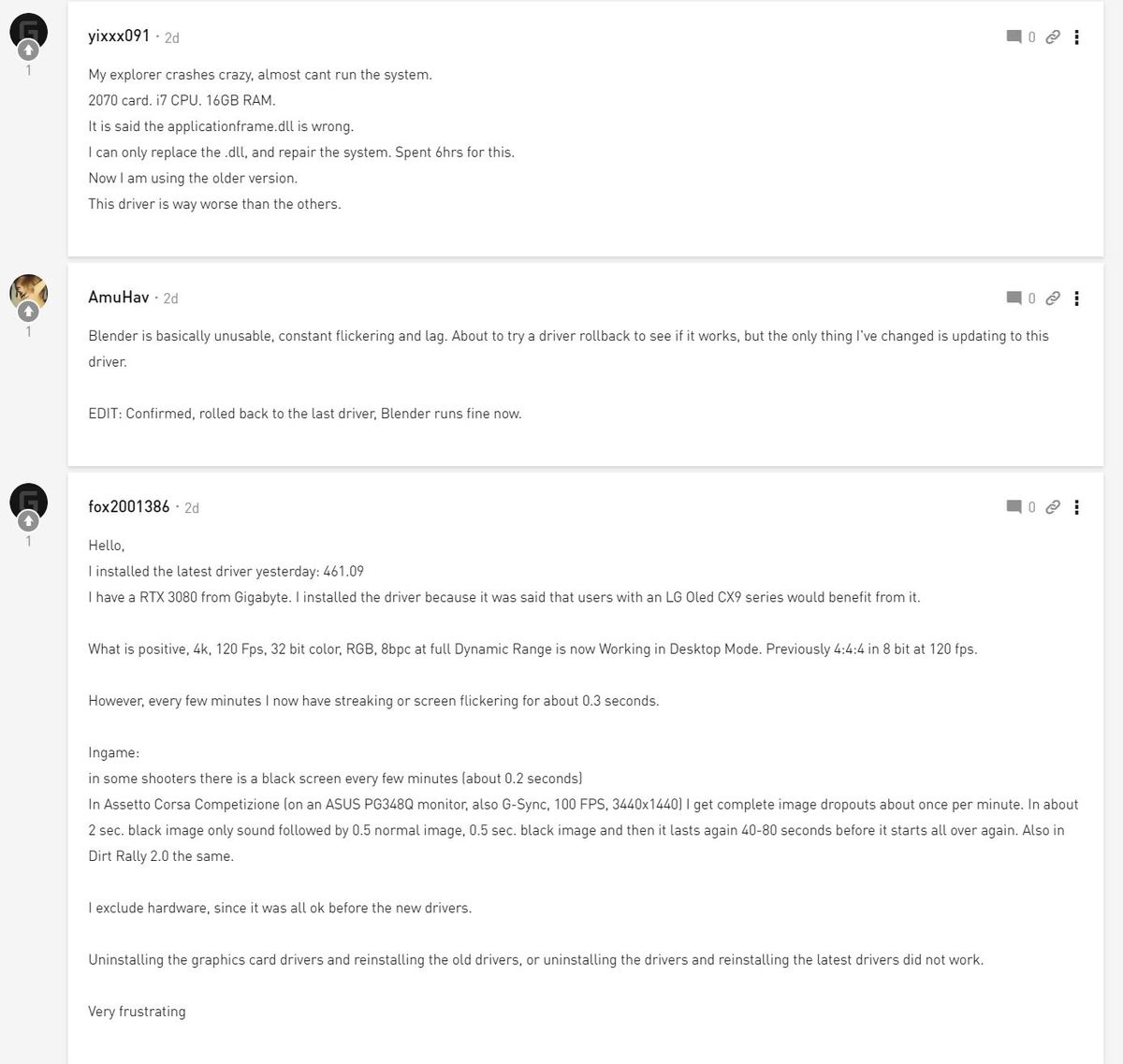In the image, we observe a screenshot of a messaging platform exchange. The conversation involves three participants, identified by their usernames and avatars at the top of the interface. The primary message, possibly from the user initiating the conversation, states: "My explorer crashes crazy, almost can't run the system." This indicates a discussion about technical issues, likely related to computer gaming, given the context and terminology used.

The replies come from two other users, "AmuHav" and "Fox2001386," who are participating in the troubleshooting conversation. The interface also features a panel on the right-hand side, including an attachment button that allows users to upload images or files, further facilitating the discussion.

Overall, the screenshot captures a dynamic and technical exchange among users, who are collectively addressing a problem experienced by one of them, likely within a computer gaming or tech-focused community.